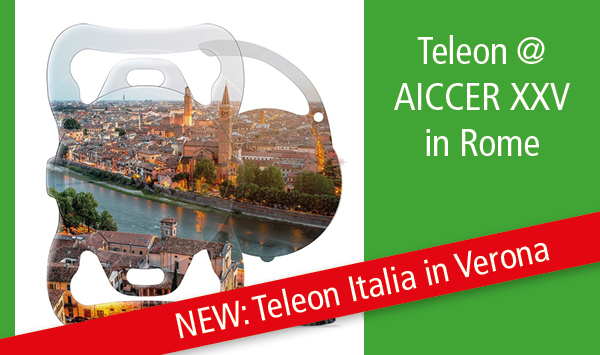The image, likely a poster or a page from a travel magazine, features a distinct layout with a white background and multiple design elements. On the left side, there is a green stripe, while the right third of the image is dominated by a green box. This green box contains white text reading "Talon at Acer XXV in Rome." Adjacent to the green box, in the white background, there is an intricate cutout shape housing a visually detailed photo of a cityscape. The city depicted appears to be Rome, featuring a waterway with buildings lining the shoreline. Above this scenic image, a red banner slants diagonally from the bottom left to the upper right, displaying white text that reads "New: Talon Italia in Verona." The overall design blends both textual and visual elements to create a compelling narrative about cities in Italy.